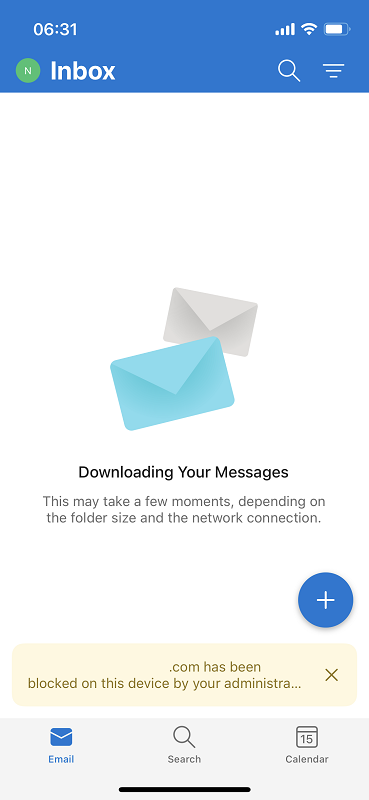This is a detailed screenshot of a smartphone inbox at 06:31. The battery is fully charged, and the Wi-Fi is connected. The interface displays a green box labeled "Inbox" at the top, accompanied by a search icon and a menu represented by three horizontal lines arranged in the shape of a pyramid. Below the header, there are two envelope icons—one white, one teal—indicating ongoing message downloads. A message beneath these icons states, "Downloading your messages. This may take a few moments, depending on the folder size and the network connection."

Further down, there's a notification reading, ".com has been blocked on this device by your administration," suggesting a restriction set by an organization, presumably the Ministry. A plus sign is also visible for adding new items. 

At the bottom of the screen, there are three navigation tabs: Email, Search, and Calendar, with the Email tab highlighted in blue, indicating active selection. The screenshot captures the inbox page as messages are being retrieved, highlighting the process and status of the email application.